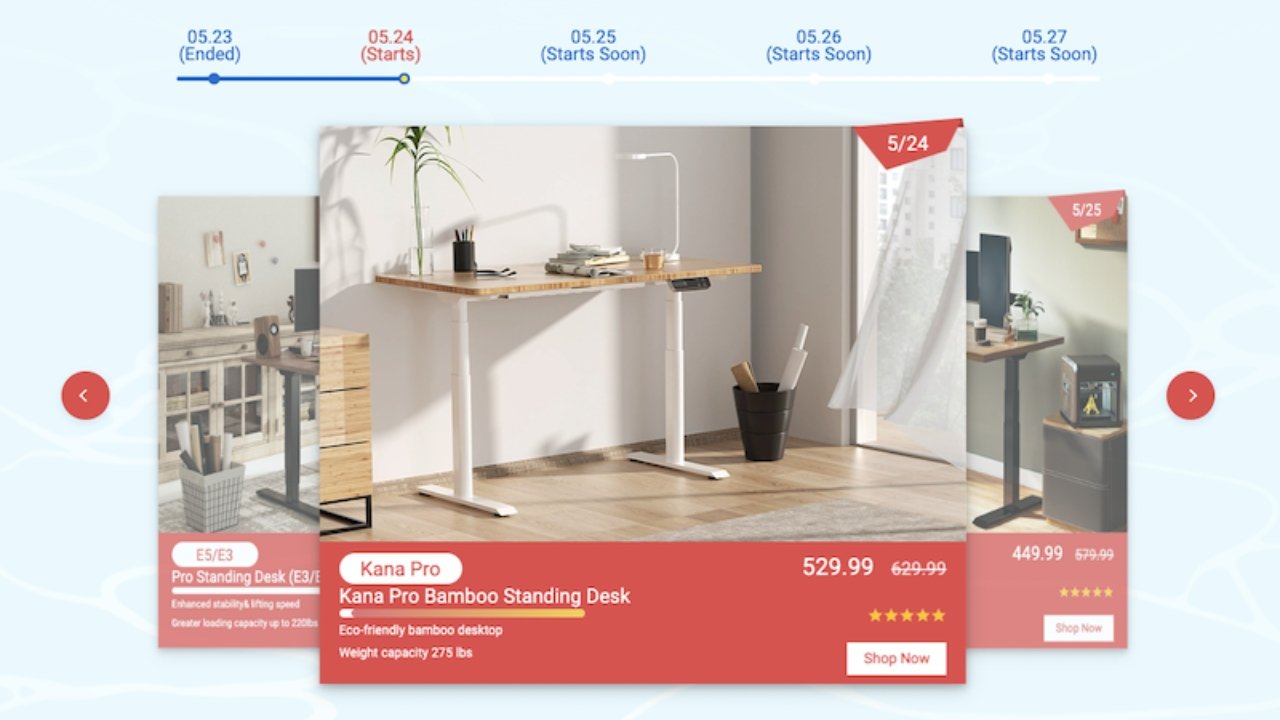The website features a light blue background with white lines scattered across it. At the top, in blue text, "05.23" is marked with the status "(ended)," accompanied by a horizontal blue progress bar against a white background. The bar is partially filled in blue up to a red marker that indicates another event, "05.24 (starts)," where the blue section ends. Subsequent dates, "05.25," "05.26," and "05.27," are listed below as starting soon.

Beneath the progress bar, there is a stack of product images. The top image showcases a stylish desk setup against a white wall. The desk itself has a wood-brown and white surface. Underneath this image, in red text, is the brand name "Kanabro," followed by "Kanabro Bamboo Standing Desk." The desk is priced at $529.99, discounted from its original price of $629.99. A "Shop Now" button in white text on a red background is also visible.

Partially obscured by the top image are other products, one of which seems to be another desk priced at $449.99, also featuring a "Shop Now" button in red. The specific details of these other products are not fully visible due to the overlapping images.